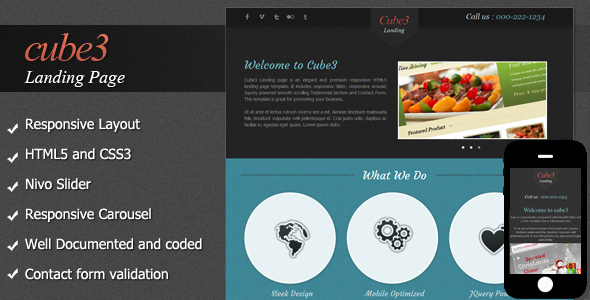This image is a detailed screenshot from a website showcasing a dark gray-themed layout. Dominating the left side is a vertical menu with a top black banner, serving as a simple rectangular header. In this banner, "cube3" is notably written in red lowercase letters, with "cube" and "3" conjoined without any space. Below this, in white text, it reads "landing page," indicating the primary function of the template.

The white-font menu items listed on the left include:
- Responsive Layout
- HTML5 and CSS3
- Nivo Slider
- Responsive Carousel
- Well Documented and Coded
- Contact Form Validation

These features suggest this screenshot represents a versatile website theme, intended for potential buyers to preview the design and functionality.

The upper portion of the main content area is bordered by a black top border, transitioning into a very dark gray, almost black, header background. Here potential users are encouraged to place a prominent photograph on the right side. In this example, there is a close-up image of a colorful salad with a mix of red, green, and yellow peppers.

On the left side of the image, against the dark background, the words "Welcome to cube3" are written in blue. The text immediately beneath this is not quite legible in the screenshot. The lower half of this section features a pleasing blue-gray shade. Within this area are three circles, which typically could serve as placeholders for icons or additional imagery.

In the lower right-hand corner, there is a rendered image of a smartphone displaying the website, meant to showcase the mobile-responsive design of the template and offer an idea of its appearance on a mobile device. This image comprehensively illustrates the layout and stylistic options available to users through this website template.